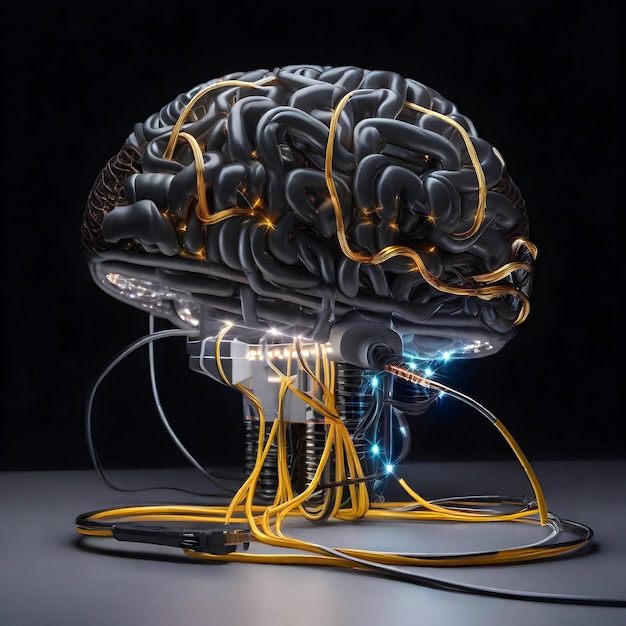The image depicts an artistic, 3D representation of a human brain that strays from anatomical realism. The brain, rendered in dark gray or black, is entwined with an array of wires, primarily yellow with some black and gray accents. These wires intertwine and connect at various points on the brain, evoking the appearance of both conduits feeding into and lines emanating from the neural mass, much like the intricate connections of a computer system. The base of the brain shows additional yellow wires, accompanied by blue and white lights suggesting active electrical currents. These connections rest upon a stand that appears integral to the structure, as if it powers or supports the brain's functions. Overall, the image appears to be a commentary on the interface between human cognition and technology, with approximately fifteen yellow wires bridging the gap between the brain and its external support apparatus.